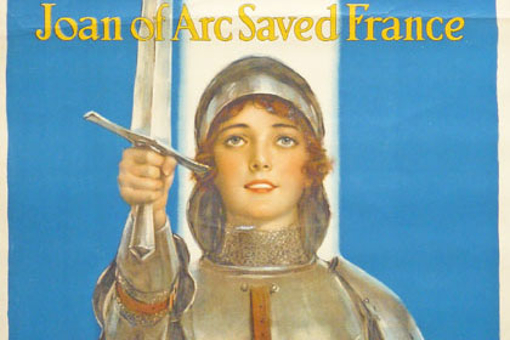The image depicts a detailed drawing or painting of Joan of Arc, identifiable by the yellow lettering at the top that reads "Joan of Arc saved France." The composition appears to be an advertisement or an old poster, rectangular in shape. Joan of Arc stands prominently in the foreground, encased in silver armor with some brown leather details adorning the front and her right arm. She has short, reddish-brown hair, blue eyes, and a complexion suggesting she might be wearing makeup, including lipstick and blush. In her right hand, she firmly grasps a silver sword raised upwards, although the hilt and tip are not visible, extending beyond the frame. Notably, her gaze is directed skyward. The background is predominantly light blue, indicating a possible sky setting, with a thick, vertical white stripe running from top to bottom behind Joan's head, serving to center and highlight her face.